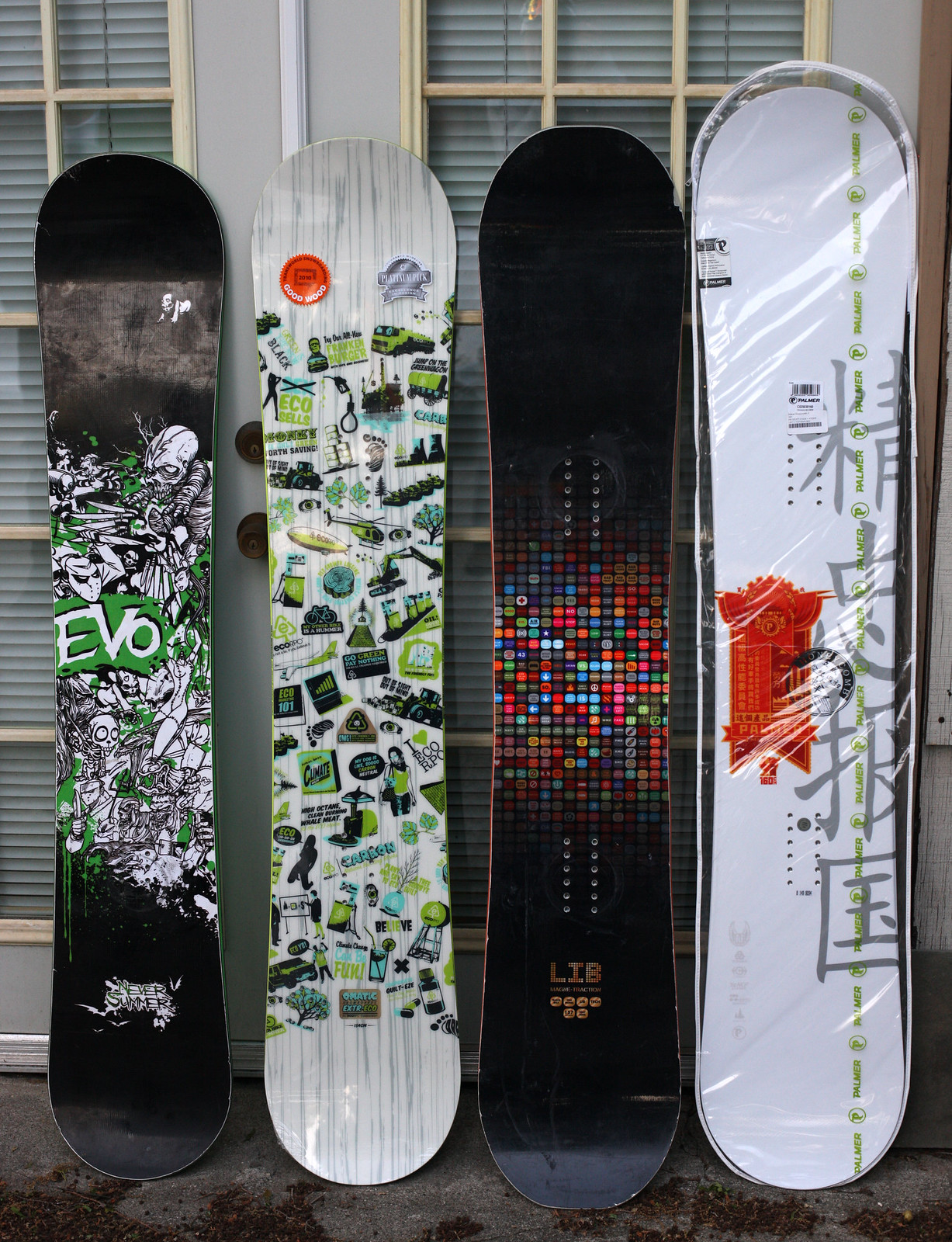In front of paned windows with horizontal blinds, likely on the side of a house, stand four vertically oriented longboards displaying distinct designs. The board on the far left is predominantly black, featuring a central white design with skeleton motifs, and the word "EVO" in a green box with white writing. At the bottom of this board, there is also a white area with black writing that reads "Never Summer." The second board from the left has a whitewashed background with intricate illustrations depicting various forms of transportation such as a helicopter, blimp, bicycle, car, train, and truck, alongside natural elements like trees. This board also contains the phrase "Echo Bells" and a recurring "eco" theme, possibly indicating an eco-friendly brand. The third board showcases a black background adorned with vibrant, neon-colored squares in red, blue, yellow, and green. Down the middle of the board runs a series of small white dots, giving the appearance of lights. The word "Lib" can be found at the bottom, in gold lettering accompanied by gold circles. The far right board is white with Asian characters and a prominent red banner-like section, suggesting an oriental theme. All four longboards, appearing lengthy without visible wheels, lean against the wall and rest on a dark ground surface, under the clear sunlight.